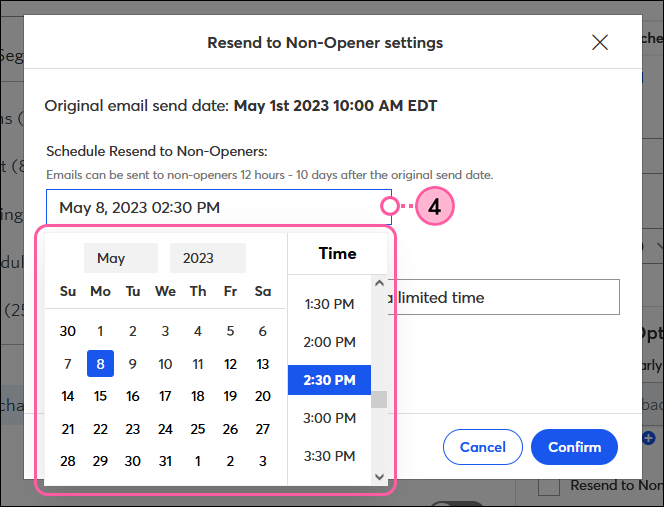This image is a screenshot captured in portrait mode. It features a highlighted section in pink, drawing attention to a pop-up form within a mail program's interface. The background, which is gray and slightly blurred, has partially legible text including segments like "SEG" at the upper left, "CHIA" in the bottom left, and "CHE" in the upper right. The bottom right shows a faint open check mark, the word "resend," and a "+" button above it.

The central feature of this image is a white pop-up form titled "Resend to Non-Opener Settings" at the top. Below the title, the form displays the original email send date as "May 1st, 2023, 10 a.m. Eastern EDT" in bold black text. The next section explains that emails can be resent to non-openers 12 hours to 10 days after the original send date, indicating that this is an automated process to target recipients who did not open the initial email.

Highlighted in the center of the form, a blue input box shows that a new resend date has been scheduled for "May 8th, 2023, at 2:30 p.m.," exactly one week after the original send date. Surrounding this input box is a pink circle, emphasizing the scheduled resend details and how to select the date using the calendar. At the bottom right corner of the form, a blue button labeled "Confirm" is visible, indicating the next step to finalize the rescheduling of the email.